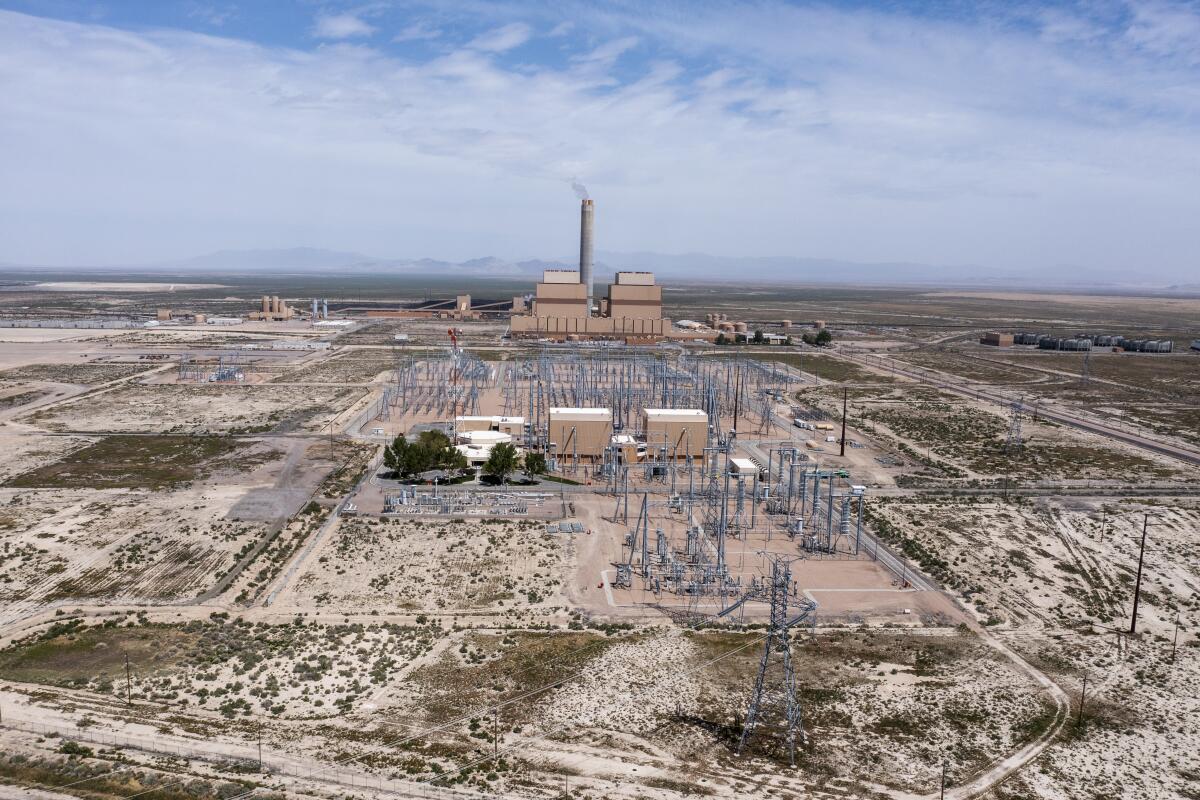This image features an expansive aerial view of a large power plant situated in a desolate, desert-like area characterized by sandy, tan-colored soil interspersed with small, brown and green scrub brush. Dominating the scene are two light brown towers marked by dark brown stripes and topped with white utility boxes, alongside a prominent gray concrete smokestack emitting smoke into the sky. The backdrop includes several large conveyors seemingly transporting coal into the burning towers, hinting at the plant's coal-based operations. To the left, a series of small air scrubbers are visible, contributing to the plant's emission control efforts. In the foreground, an extensive power station bristles with numerous metallic poles and towers, housing two substantial power diversion boxes and a small trailer functioning as an office. The utility structure is complemented by rows of large power lines and substations. The surrounding region appears particularly barren, with no additional structures in view, highlighting the isolation of the plant. Beyond this industrial expanse, a lofty mountain range stretches across the horizon under a vibrant blue sky adorned with bright white clouds and some wispy, overcast patches, contributing to the scenic but remote setting of the power plant.